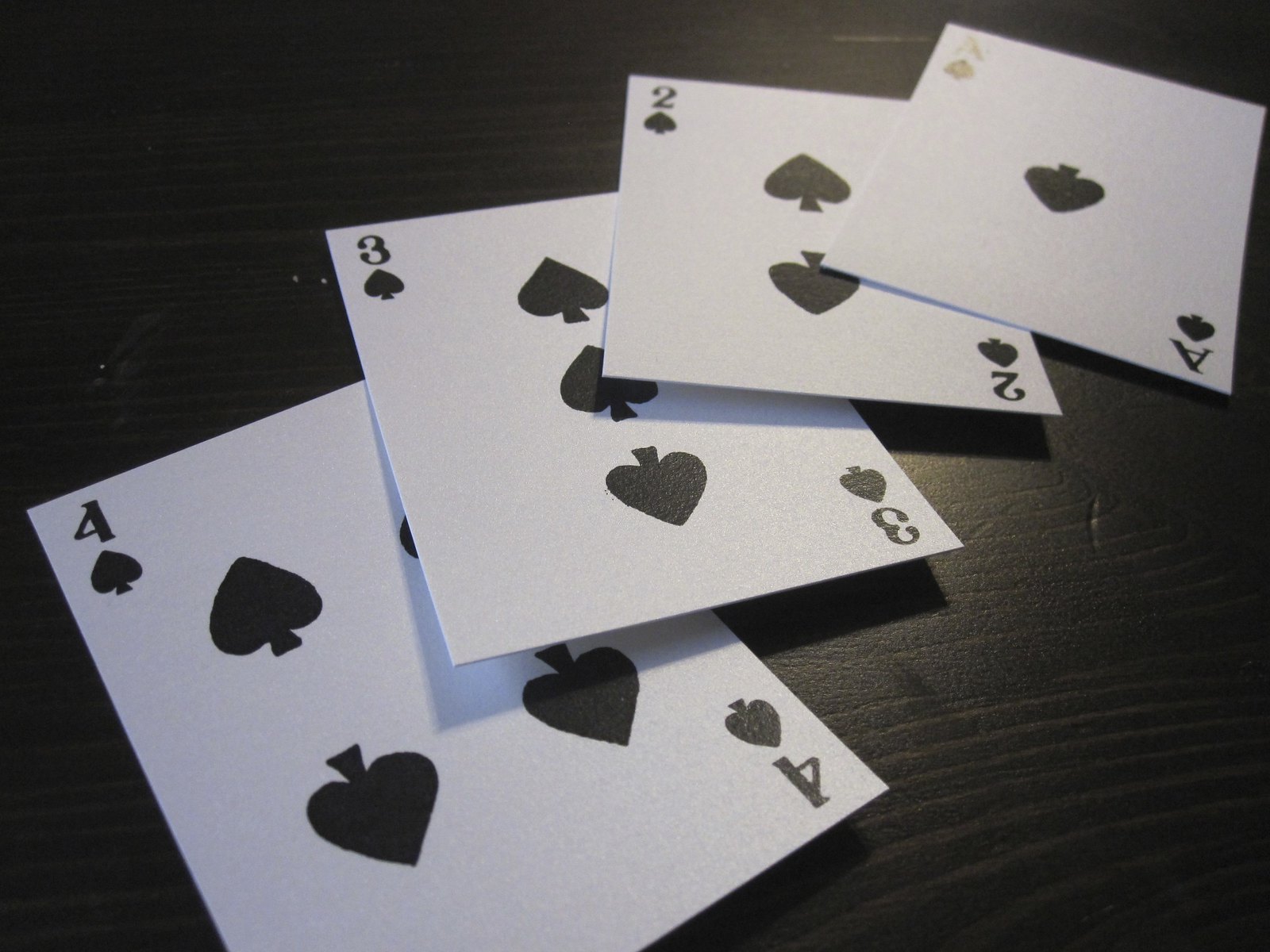This photo features four meticulously arranged playing cards placed on a textured black wooden surface. The wood grain is distinctly visible, showcasing lighter lines that contrast beautifully against the dark background, adding depth to the scene. Each card is stark white, adorned with black spades and sharp, angular corners. 

From bottom to top, the cards are arranged as follows: 
1. The four of spades, characterized by the numeral '4' in both the upper left and lower right corners, each accompanied by a petite black spade. Four larger, prominent spades occupy the center of the card.
2. The three of spades, slightly overlapping the four of spades. Similar to the previous card, it features the numeral '3' in the upper left and lower right corners, with a small spade underneath each. Three larger, centered spades complete the design.
3. The two of spades, continuing the overlapping pattern. This card displays the numeral '2' and small spade placement identical to the others, with two large spades in the center.
4. The ace of spades, crowning the arrangement, showcases a prominent capital 'A' in both corners, each accompanied by a small spade. At its center stands a single, inverted large black spade, acting as a striking focal point.

The composition of the image, combined with the contrast of the cards against the dark wooden surface, creates a visually compelling and detailed representation of this classic card sequence.